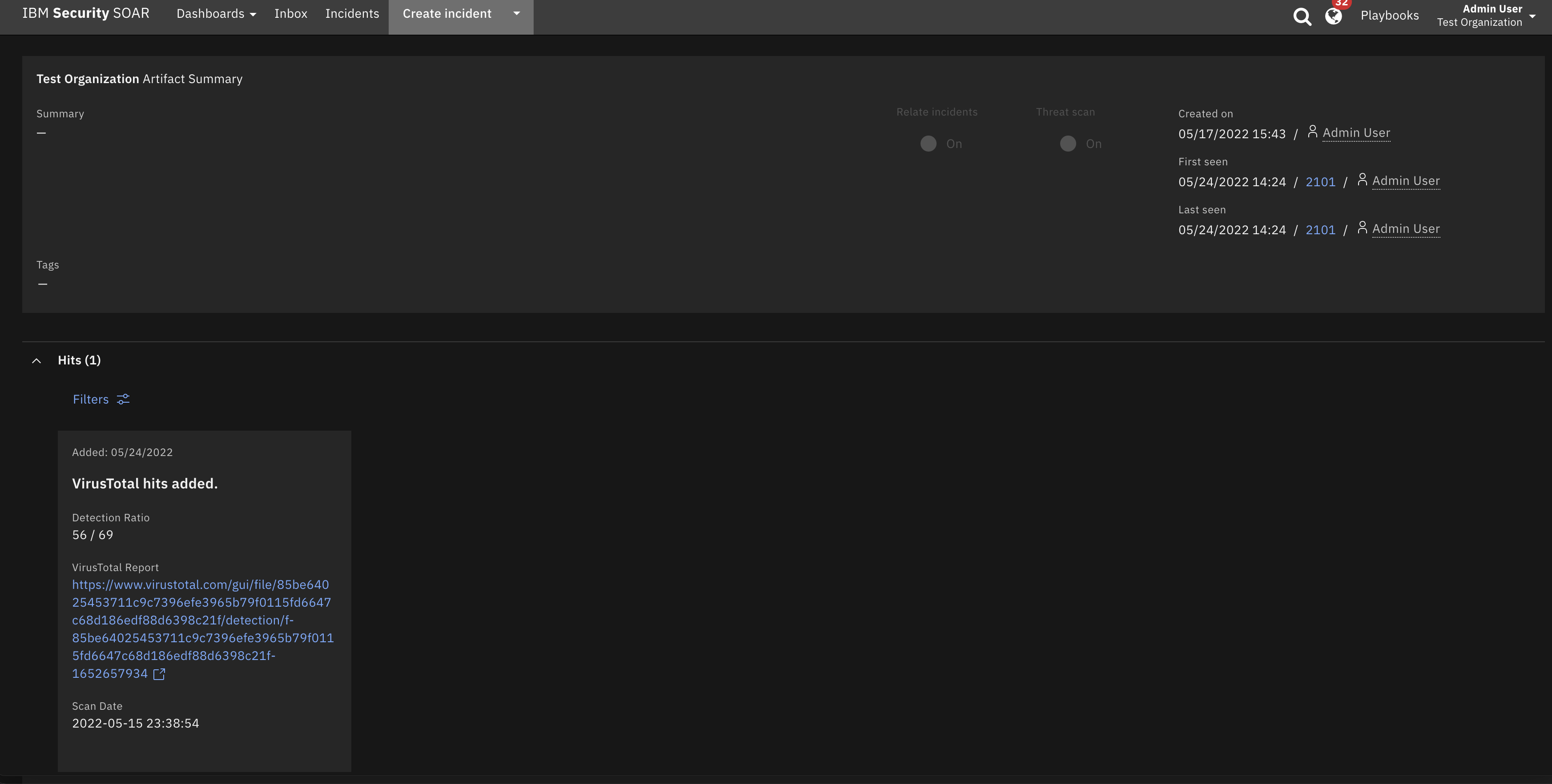The image depicts a black-themed website interface, primarily focused on security. On the right side, adjacent to the search bar, there is a noticeable red circle with a white number inside, indicating notifications. The left side prominently features the heading "JBM Security Test Organization." Below this heading, details are quite minute and hard to decipher. There appears to be a reference to "virtuous total" which is highlighted in white, and several lines of text written in blue. The right side of the page also contains numerous white lines interspersed with some blue text, but this text is too small to read clearly. In the upper-left corner, the menus include options for "Dashboards," "Inbox," "Indents" (though this may actually be labeled differently), and "Create” something, potentially "Create Indent." Additionally, in the upper-right corner, there is a section that seems to be labeled "Playbooks," but the tiny font size renders most text largely unreadable.